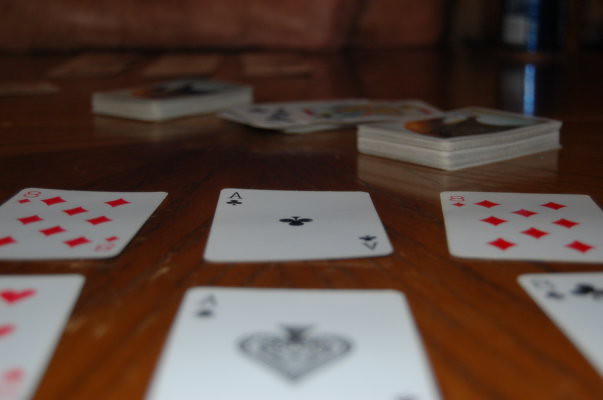This photograph captures an eye-level view of a dark, scratched wooden table scattered with playing cards. At the center of the composition, in sharp focus, lie an ace of spades and directly above it, an ace of clubs. To the left center, an eight of diamonds is clearly visible, mirrored by another eight of diamonds to the right center. In the lower right corner, an out-of-focus eight of clubs can be spotted, while the lower left corner reveals a partially visible, blurred hearts card. The bottom edge of the photo is notably blurry, creating a depth-of-field effect that contrasts with the slightly out-of-focus background. Three decks of cards are positioned in the background; two are precisely stacked and face down, while the middle deck is slightly disheveled with some cards face up and fanned out.